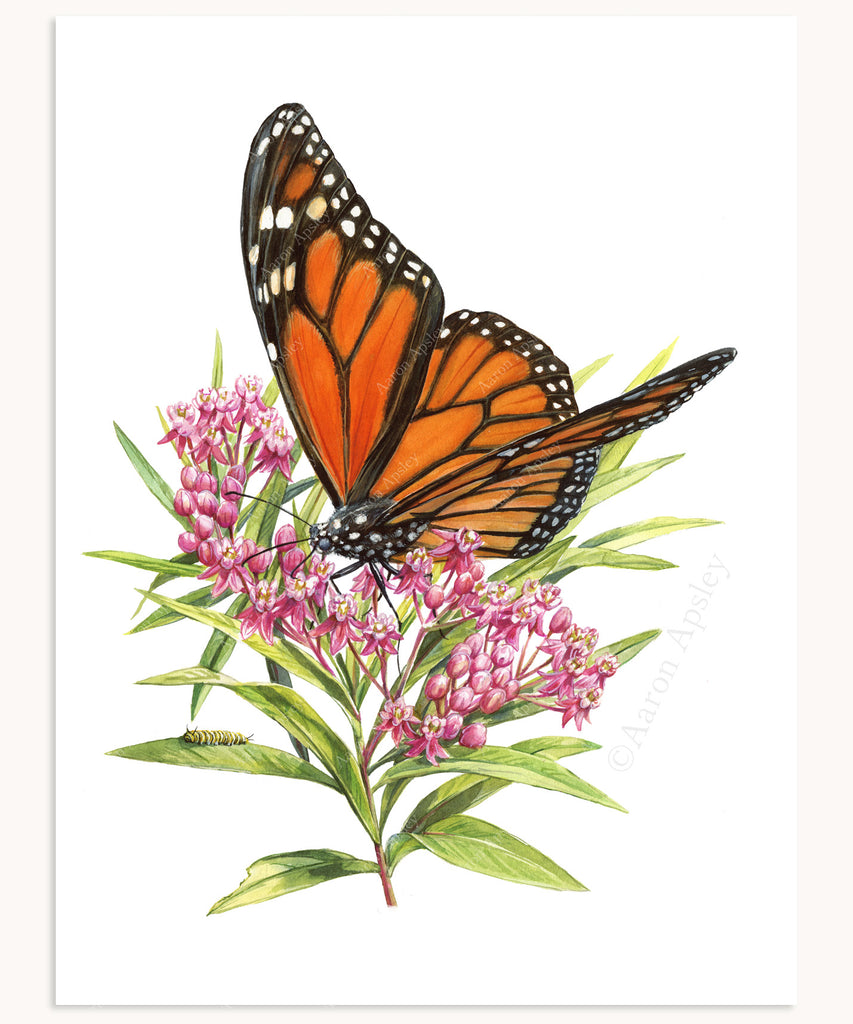This image depicts a lifelike, hand-drawn artwork, likely created with colored pencils. It features a majestic monarch butterfly poised on a cluster of delicate, light pink flowers with vibrant yellow centers. The butterfly's signature large orange wings, edged with distinctive black and adorned with white spots, are spread out, showcasing its vibrant pattern. It has a black body speckled with white dots. Attached to the flowers are elongated green leaves, from one of which, on the left side, a green caterpillar - possibly the monarch's larval stage - is crawling. The background is a plain white, enhancing the colors of the butterfly and flowers. Additionally, a watermark reading "Copyright Aaron Alpsley" is faintly visible on the left side of the image.